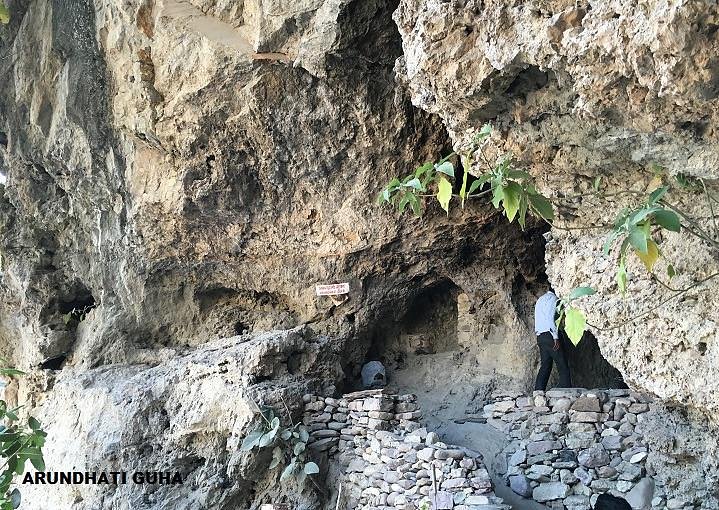This detailed outdoor daytime photograph captures a striking scene reminiscent of a tourist postcard, featuring a stone cliff with a historic dwelling area carved into it. The earth-toned cliff rises from the ground, filled with boulders and crevices that create natural walkways. On the left and right of the walkway, several stones are stacked like bricks, adding to the ancient feel of the site. The central focus is on a man, distinguishable by his dark skin tone, black pants, and a blue long sleeve shirt, who is stepping into a doorway carved into the cliff face. Flanking the entrance are windows with pottery arranged outside, showcasing local craftsmanship.

The walkway leading to the cave-like formation is covered in dirt and resembles cobblestoned paths, enhancing the rustic aesthetic. Various green branches and leaves sprout intermittently from the rugged cliff sides, adding a touch of nature's resilience to the scene. Notably, there is a white sign in the frame, though its text is too distant to decipher. Additionally, text reading "Arundhati Guha" is visible at the bottom left corner of the image. This picturesque setting, devoid of sky view, immerses the observer in the raw beauty and historical allure of the stone formation and its enigmatic dwelling spaces.